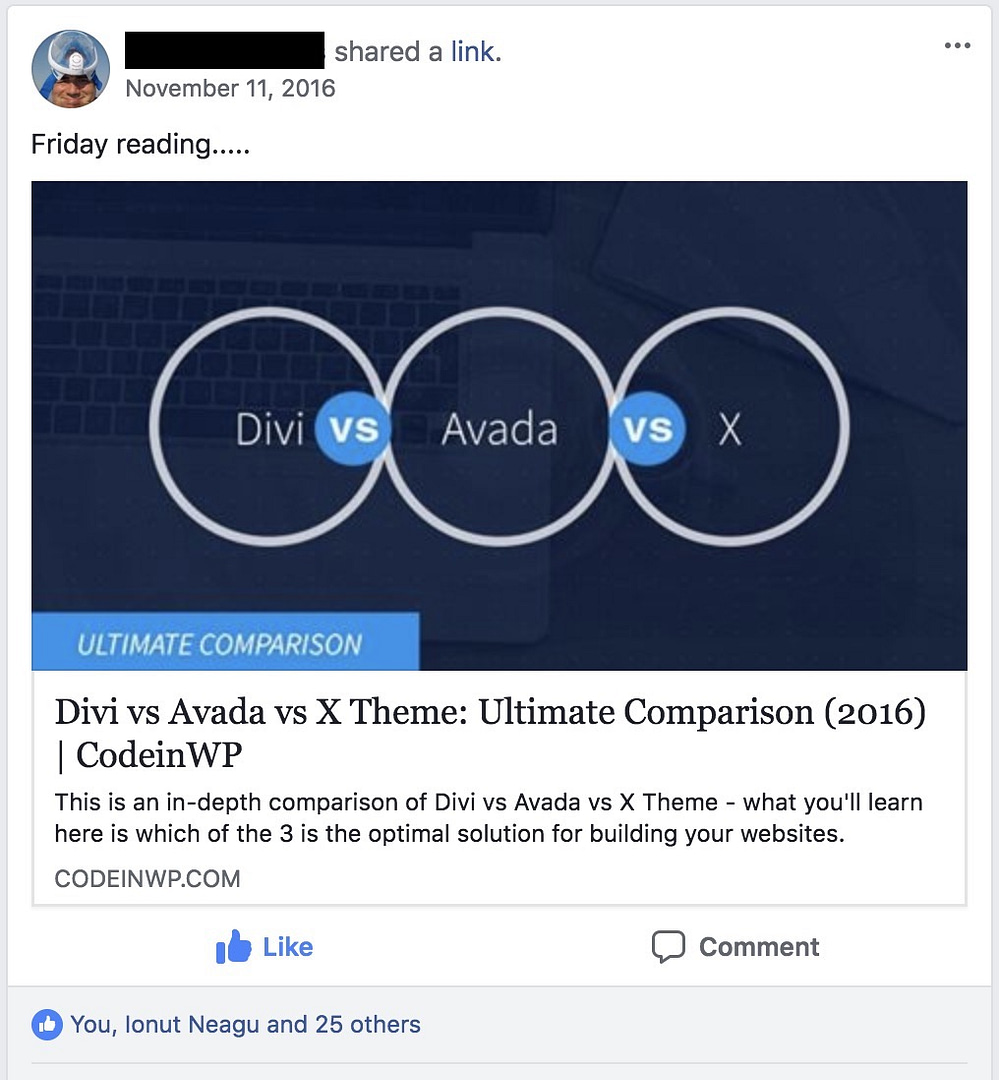This image is a screenshot from Facebook, taken on November 11th, 2016. It features an anonymized male user, whose name has been blocked out for privacy reasons, sharing a technical link on their timeline. The thumbnail photo of the user shows him making a funny face, but further personal details are obscured. The shared link is titled "Divi vs. Avada vs. X Theme: Ultimate Comparison 2016 - Code NWP," suggesting an in-depth comparison of three website building themes, aimed at helping the reader determine the optimal solution for their needs. The user added a caption: "Friday reading….." The screenshot also indicates that the post received engagement, with the person taking the screenshot and 26 others liking the shared link. The content appears highly technical, likely catering to industry professionals and experts in website development.